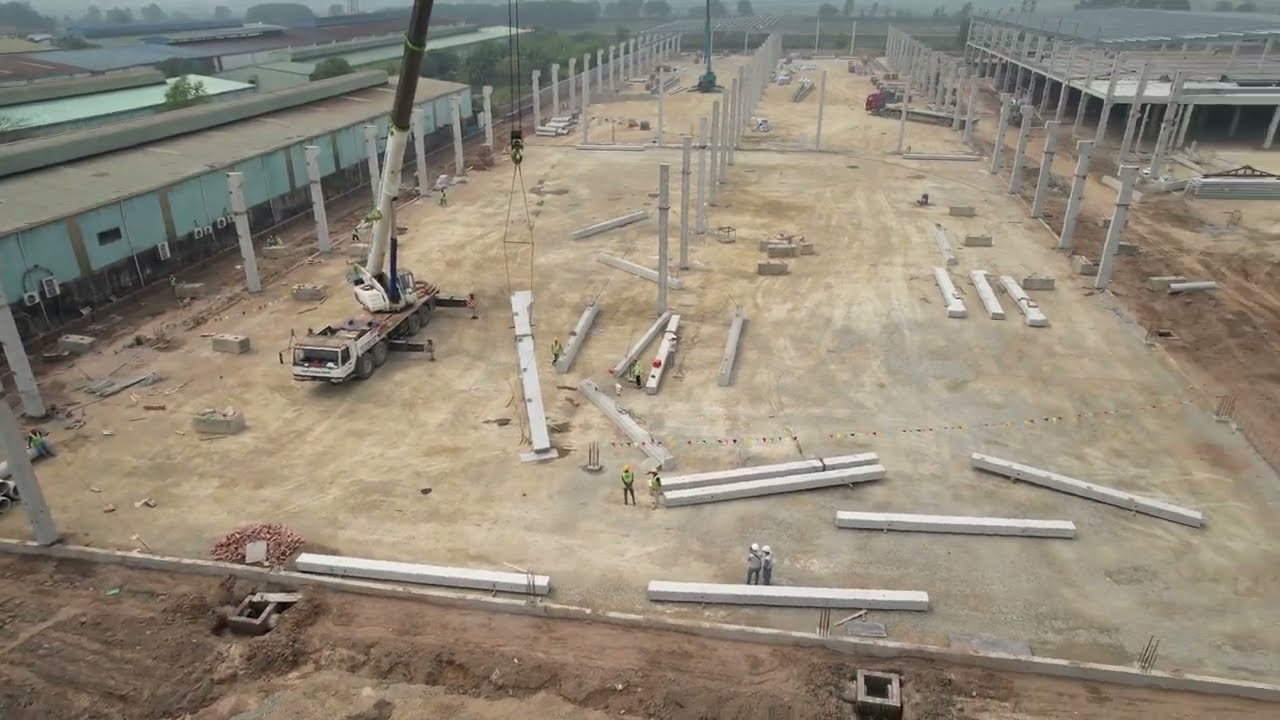The image captures a high-angle view, likely from the top of a building, a parking garage, or a drone, showcasing an expansive construction site. Dominating the scene is a crane lifting white steel columns, each roughly 20 to 25 feet tall, which are being positioned to form the foundation of a new structure, possibly a large warehouse or industrial building. The sandy, compacted soil area below is meticulously prepared for the construction effort, with several construction workers, though small in the photograph, actively engaged in the project. To the right, a light blue warehouse stands, juxtaposed against the new structure that is beginning to rise on the left. The scene is bustling with activity, from workers clad in hard hats, apparently engaged in discussions, to the methodical placement of columns by the crane, suggesting the early stages of an extensive building endeavor.